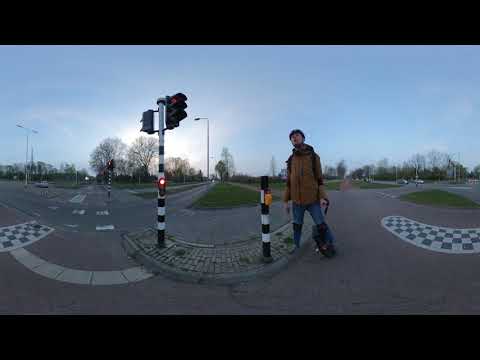The image captures a young man standing at a crosswalk in what appears to be a European street, characterized by a solid black border framing the scene. Positioned centrally within the composition, the man wears a brownish-tan long-sleeved jacket, a black scarf, blue jeans, and a helmet. He also appears to be equipped with knee pads, suggesting he might be riding an electric unicycle nearby, though the object isn't clearly visible. Adjacent to him is a distinctive black pole with white stripes, topped by a stoplight displaying a red signal. 

The surroundings feature sparse trees, likely leafless due to winter, and a couple of distant cars, enhancing the impression of a fairly empty street. There is also another black and white pole and a bike path or secondary street intersecting the scene. The sky above is painted a clear light blue, signifying daytime with minimal clouds. The overall atmosphere is that of a tranquil, outdoor urban setting, possibly approaching the early evening as hinted by the softly illuminated sky.